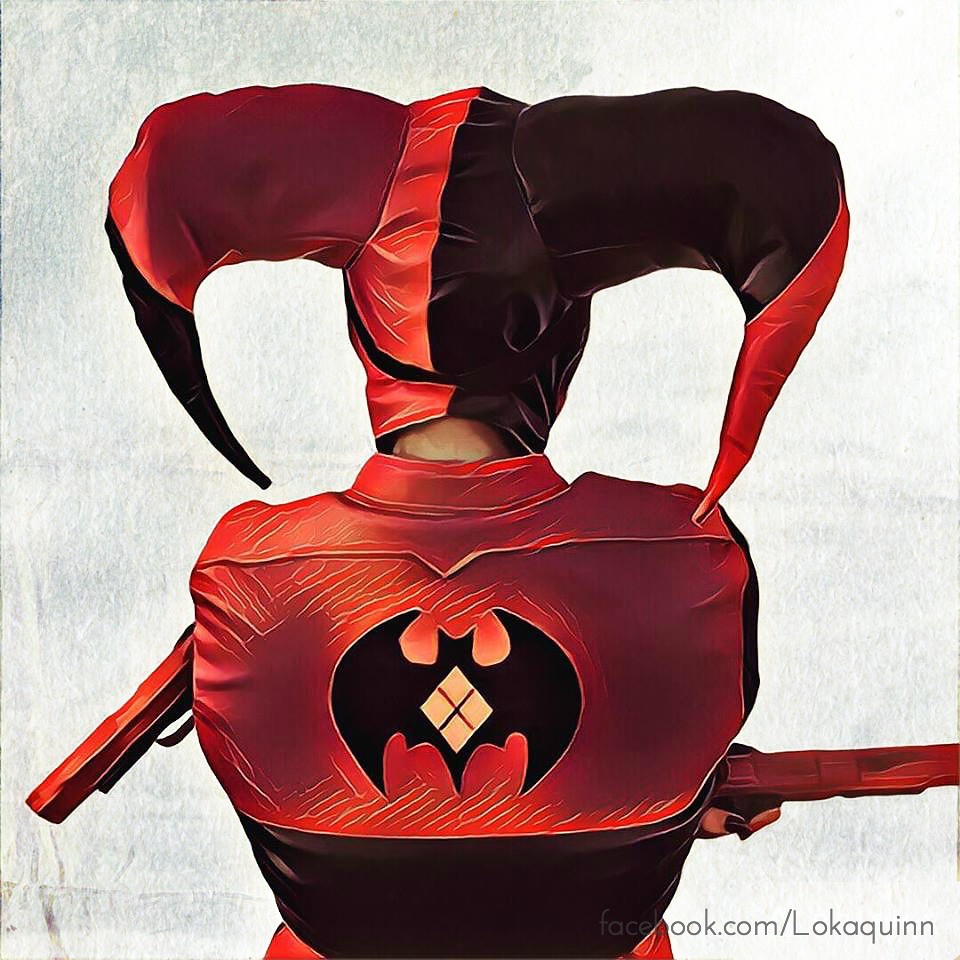The image showcases a vivid digital artwork set against a grey backdrop, depicting a solitary figure standing with their back turned. The figure is striking a powerful pose with arms crossed, each hand brandishing a gun, visible from either side. The outfit they wear is predominantly red, accented by a black waist belt. Emerging from beneath the belt, the red fabric continues seemingly uninterrupted. Adorning the person's head is a distinctive jester hat, split into red and black halves, each tipped in the opposite color. A striking feature of the ensemble is the bat silhouette on the back, highlighted by an orange diamond at its center. The lower right corner of the image bears the text "facebook.com/locaquin," hinting at the artist's social media presence.